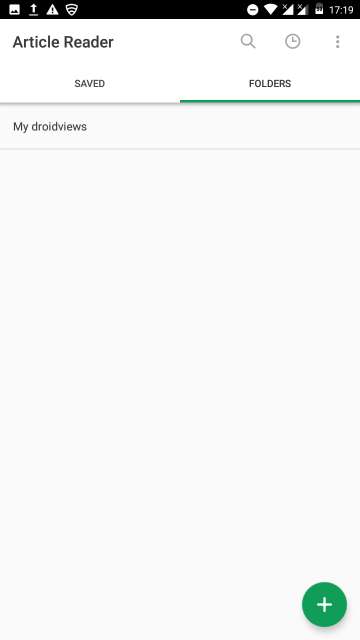This screenshot from a smartphone displays a page with a white background and a black top border. At the top left, the time is shown as "17:19" in a 24-hour format. Adjacent to the time, there is a battery icon indicating that the battery is approximately half charged. Following the battery icon, there are two icons for wireless connection and an icon for Wi-Fi connectivity. Next to the Wi-Fi icon, there is a white circle, which seems to be an ambiguous notification.

On the left side, there are several notification icons. The first is a white square, followed by an upward-pointing white arrow. Next to the arrow is a white rectangle with a black exclamation mark, signifying a warning message. The fourth icon is an inverted triangle outlined in white, featuring curving lines.

In the main section of the page, "Article Reader" is written in grey font at the top. Below this, on the left side, it reads "Saved," and on the right side, it says "Folders." Further down, on the left, it reads "My Droid Views." The rest of the page appears blank, except for a green circle with a white plus sign located in the lower right-hand corner.